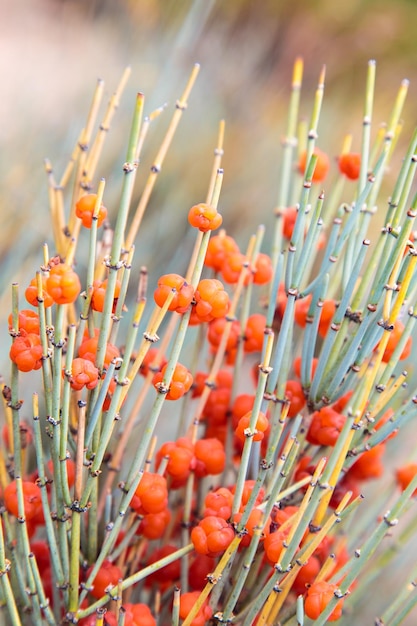The image depicts a collection of plants with long, slender stems that range in color from green to yellow to pink. Each stem features small, round protrusions that resemble berries or flower buds, varying from light orange to bright red. These protrusions are scattered along the stems, sometimes below or above each other, adding a textured appearance to the plant. The stems have no additional branching. In the background, the image is blurry, presenting a blend of indistinct colors that emphasize the sharp focus of the plants in the foreground. The overall scene captures the intriguing and colorful details of the plants against an unfocused backdrop, contributing to an almost surreal or potentially fabricated visual experience.